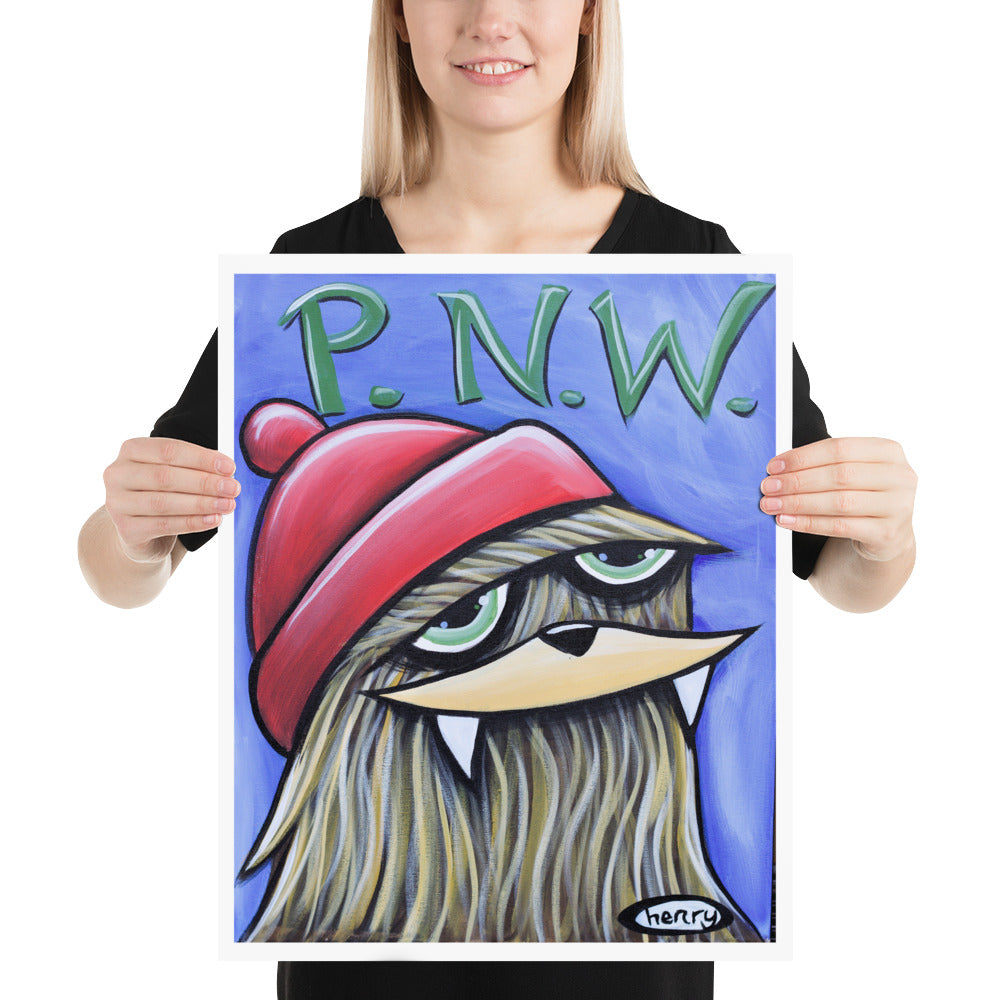The image features a young woman with straight blonde hair that falls behind her shoulders. Dressed in a black top with elbow-length sleeves, she holds a large, vertically-aligned rectangular sign in front of her chest and waist. Her hands grip the edge of the sign, and you can see just a small portion of her legs at the bottom, which are clad in black. The upper part of her face is not visible, starting from her nose down, but she has a cute smile.

The sign she is holding has a distinct design: it features the letters "P.N.W." at the top in green with a bit of white detail on each letter against a blue background. Below the text, there is a depiction of a furry, Grinch-like creature with a frowning expression. The creature has green eyes, a small black nose, white mustache turned down at the corners, and two fangs. It wears a red wool cap with a pom on the tip. On the lower right side of the painting or drawing, the name "Henry" is written and circled in black marker against a white background. 

The image is set against a solid white background, and the lighting is bright and natural, providing clear visibility.